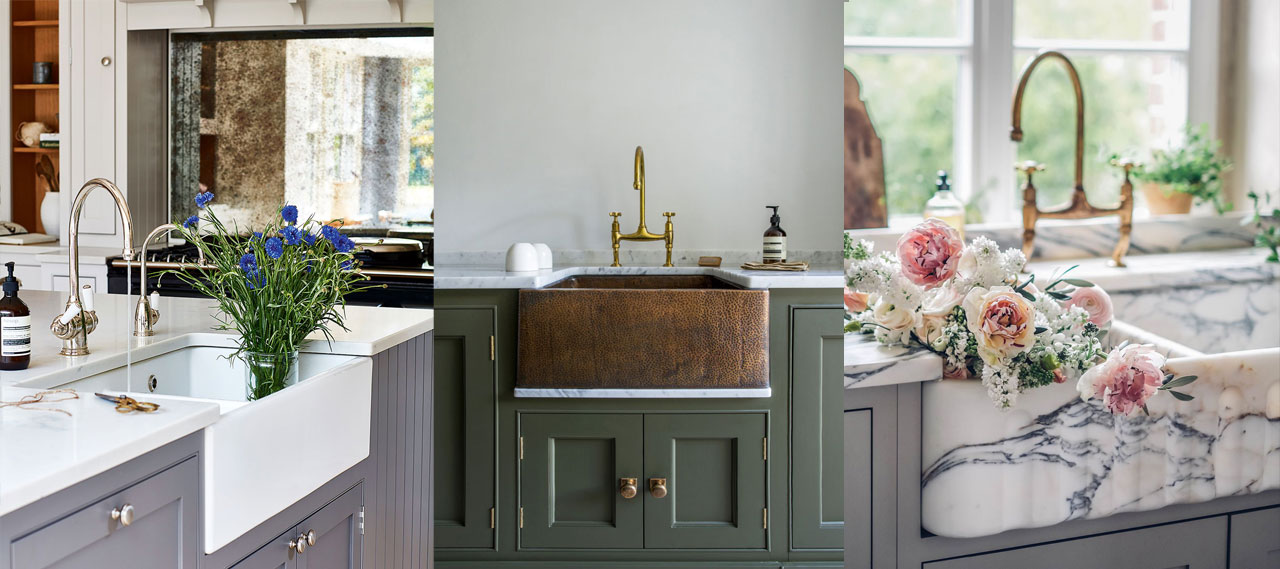The image is a collage featuring three different bathroom and kitchen setups, each showcasing a distinct sink design. On the left side, there is a bathroom sink set against light gray walls and mounted over light gray wooden cabinets. The sink itself is white porcelain with a chrome silver faucet, and a vase with blue flowers appears to sit on the countertop, suggesting they are being watered. A background view reveals more of the white-themed kitchen decor.

In the middle, the scene shifts to what appears to be another bathroom setup. Here, the cabinets below the white marble countertop are forest green. A gold-colored faucet complements the elegant design, and in front of the sink, a brown towel or leather piece is neatly placed. The walls are a clean white, enhancing the sophisticated vibe.

The right side of the collage displays another kitchen sink, this time featuring a white marble sink with dark gray marbling. The dark gray cabinets below add a striking contrast, and the gold faucet adds a touch of opulence. The background includes a window that looks out onto an outdoor scene with trees. Additionally, there are pink and white roses artistically placed on the countertop, enhancing the overall aesthetic of the setup.

Each part of the collage offers a unique yet cohesive blend of colors and materials, illustrating different styles of sinks and cabinetry, perfect for both bathroom and kitchen settings.